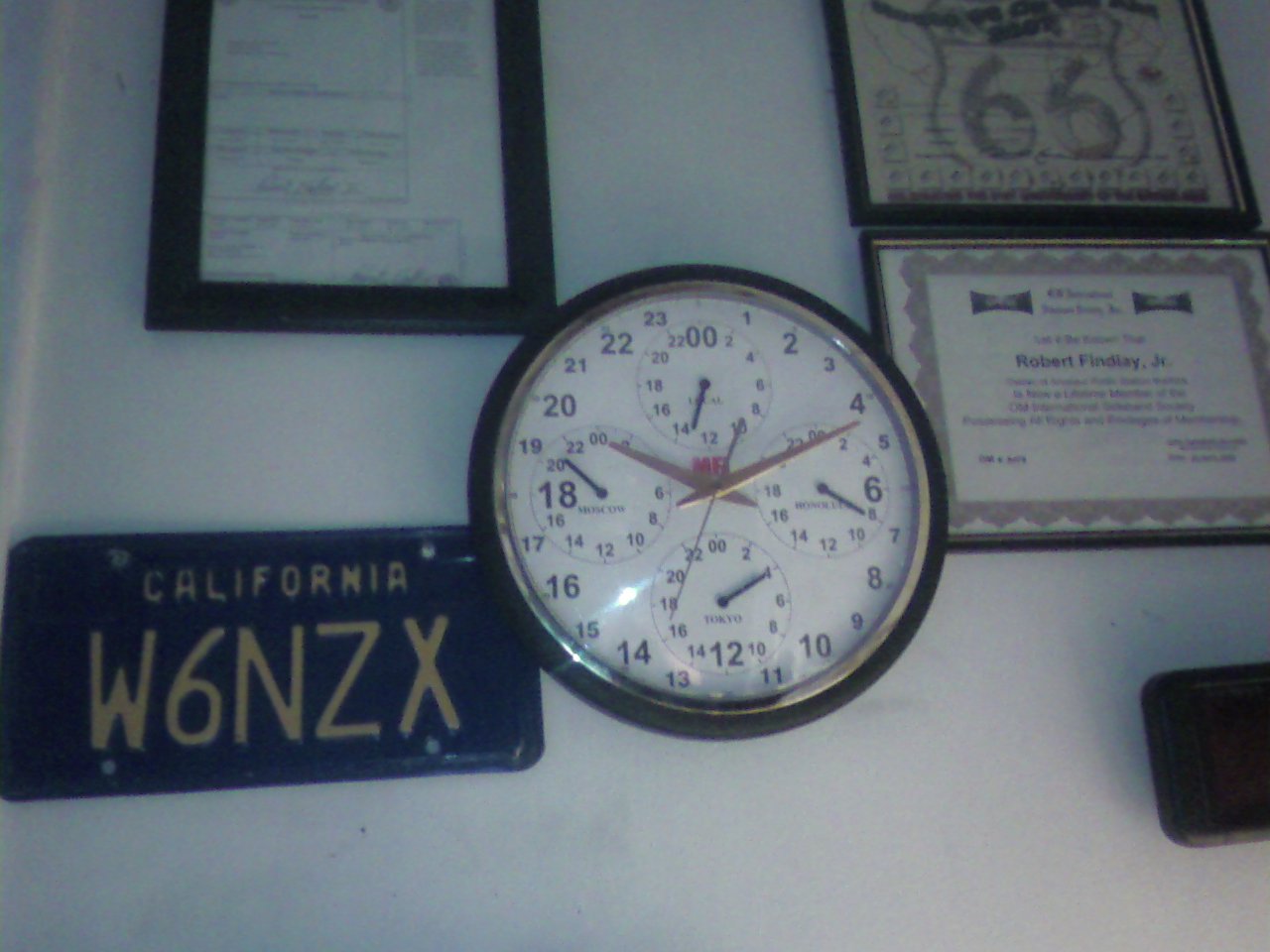This photograph showcases an eclectic array of items meticulously arranged on a pristine white wall. Dominating the upper section is a black frame containing a white piece of paper adorned with black text, prominently featuring the name "Robert Finlay Jr." and the title "Certificate of Achievement." Adjacent to it, another black frame houses a piece of memorabilia from Route 66. In the center of the composition, a clock with a black body and a white face, embellished with black numbers and several hands, commands attention. Below the clock, an antique California license plate, marked by its dark hue and golden characters, bears the registration number W6NZX. To the far right of the image, a square-shaped bronzy object adds a touch of rustic elegance to the otherwise monochromatic theme.